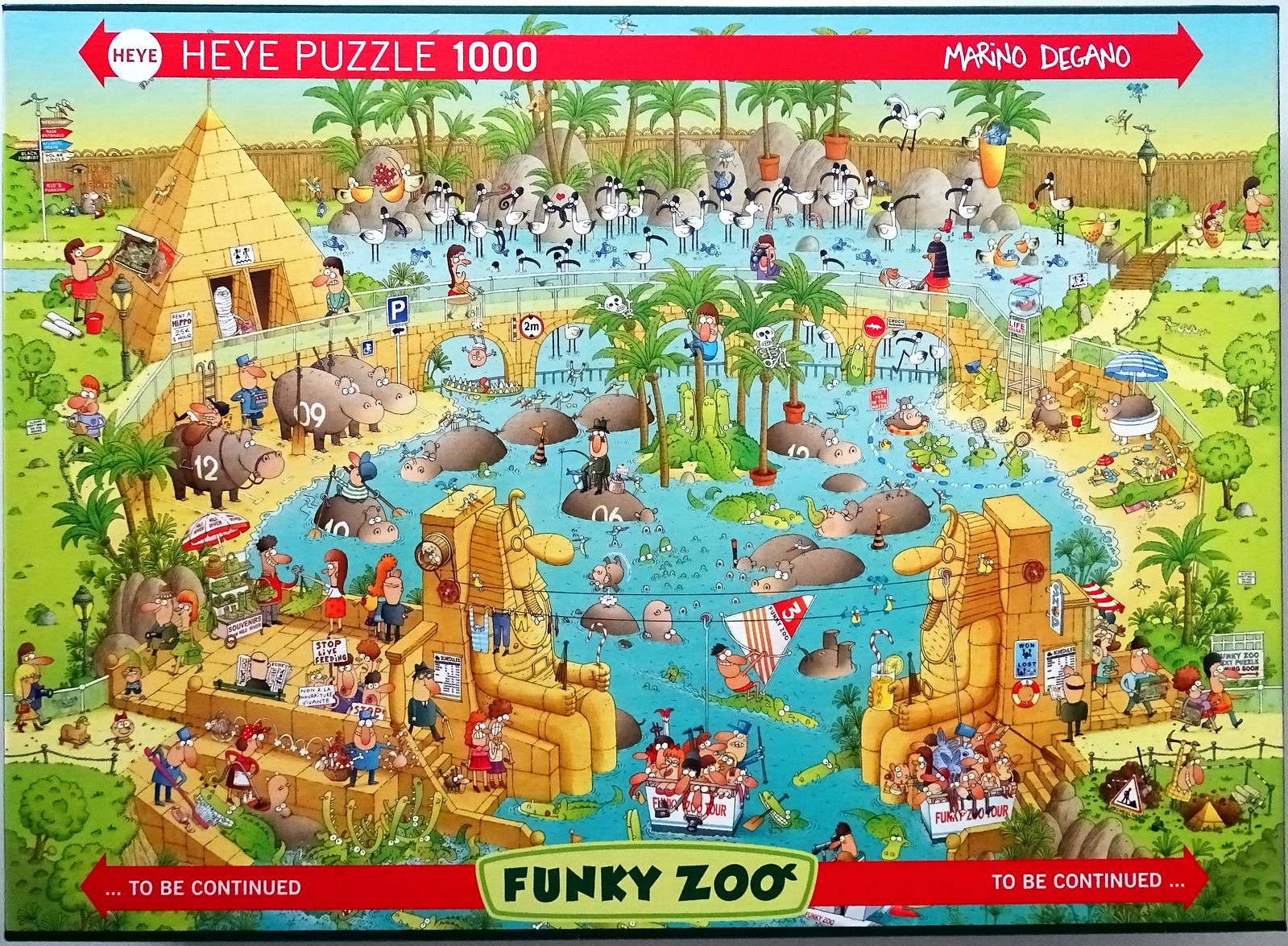This intricate "Where's Waldo?" picture, titled "Funky Zoo," bursts with vibrant, diverse colors such as blue, gold, green, red, white, and yellow. The scene is a lively medley of settings and activities: a beach teeming with hippos, majestic pyramids rising in the background, and people engaging in various activities like climbing trees. The image is a riotous celebration of both color and action, intricately designed to challenge and delight those searching for Waldo amidst the chaos.